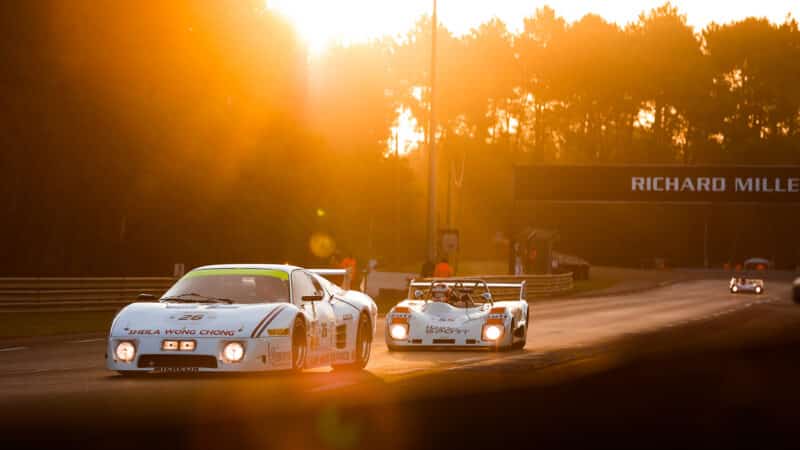The image depicts a vibrant sunset scene at a racetrack prominently featuring three white race cars. The sun is hanging low in the sky, casting an orange hue and long shadows across the track. The two cars in the forefront, sporting various sponsorship stickers and decals on their modern designs, are positioned very close to each other. The car in the lead, marked with the number 26, has a traditional sports car shape with various sponsor logos adorning its body. Closely trailing it is a more square, box-shaped vehicle that resembles a Formula One car. Both cars have their headlights on, emphasizing the dimming light conditions. 

In the distance, another white race car can be seen, slightly trailing the pair. The backdrop includes a row of trees and the silhouette of buildings, suggesting the racetrack is set in a more rural area. There's a black banner with white lettering that reads "Richard Miller" stretching horizontally across the track. Along the sides of the racetrack are guardrails and a few scattered spectators watching the race. The entire scene is bathed in the warm, saturated glow of sunset, highlighting the intense yet serene atmosphere of the race.